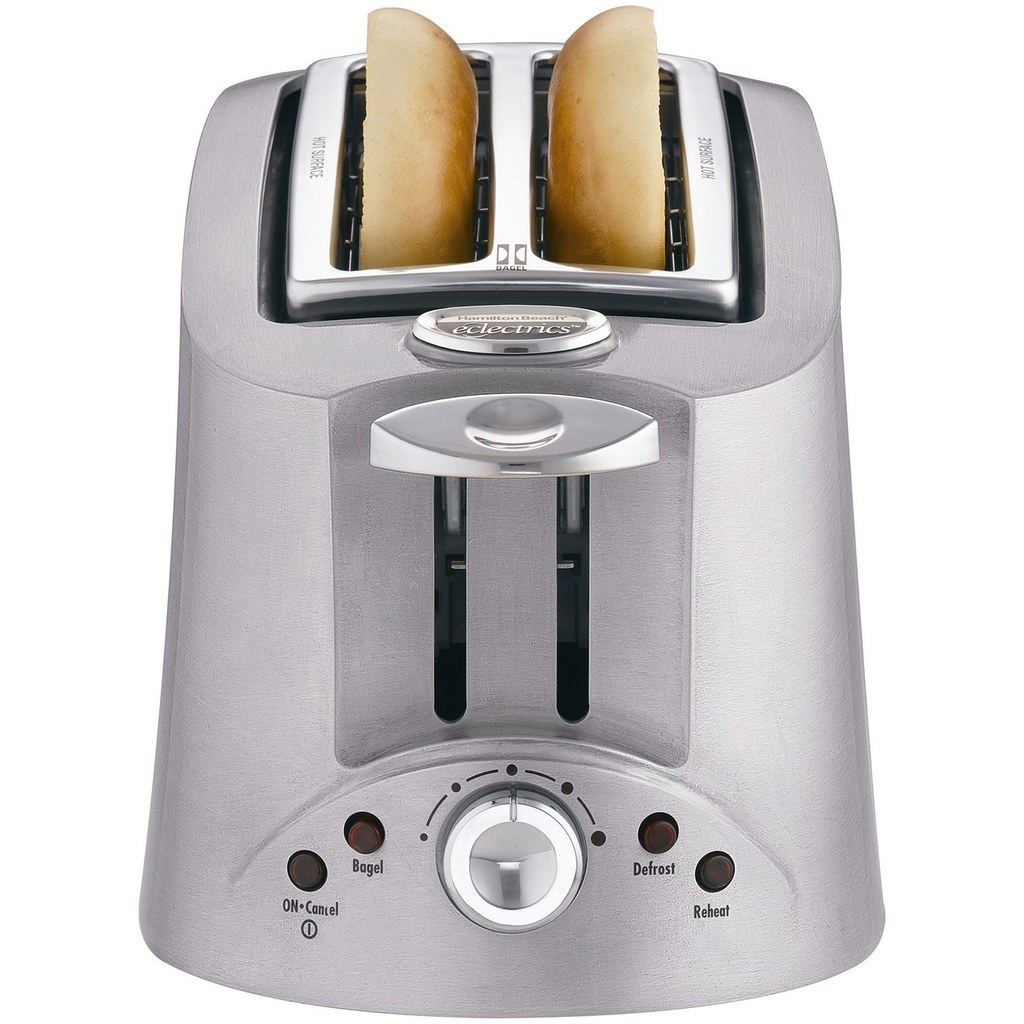This color photograph features a sleek, modern toaster in a stainless steel finish displayed against a white background. The toaster has two wide slots, each holding half of a freshly cut bagel with the browned tops facing up, ready to be toasted. The front panel of the toaster boasts a variety of controls, including an easy-to-read, round silver dial at the bottom for adjusting toast darkness, indicated by five circles that grow progressively larger. Above this dial, the control panel features four black buttons: the "On/Cancel" button on the left, the "Bagel" button above it, the "Defrost" button to the right, and the "Reheat" button beneath the defrost. A spring-loaded handle, used to push the bagels down for toasting, sits prominently above the control buttons. The brand name is identified as Eclectrics, though partially obscured by the angle. The toaster’s contemporary design is accentuated by shiny silver trim and subtle black lines.